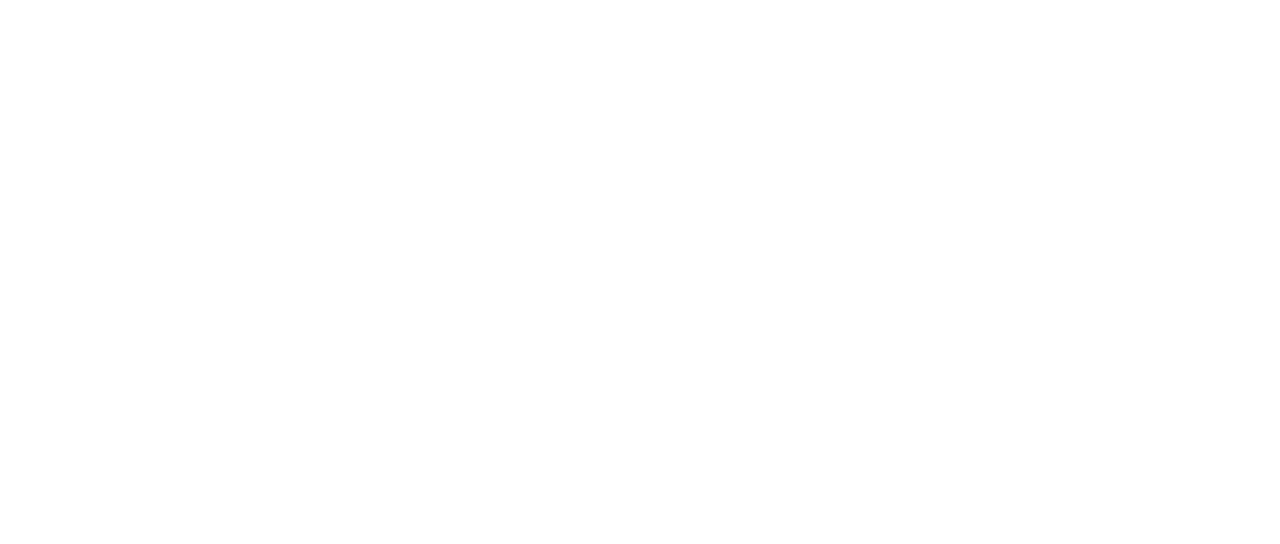The image intended to be displayed on the page has not loaded, resulting in a blank, white screen. Multiple attempts to refresh the page confirmed that no photograph or any other visual elements are present. Despite previous successful completions of similar tasks, this instance shows no objects, text, or colors other than white. There is no setting, style, or positional details to describe as the screen remains entirely blank.